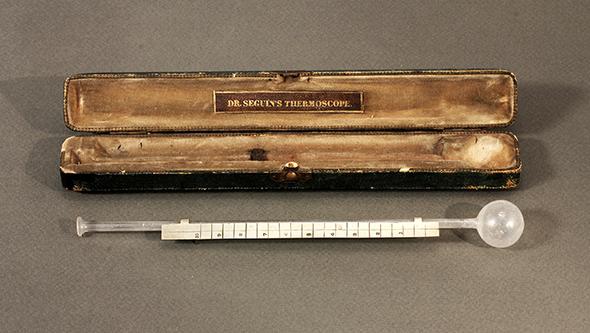The photograph showcases an antique medical instrument known as Dr. Seguin's Thermoscope. The thermoscope, a long, thin vial with a bowl-shaped end, is made of glass and lies flat on a gray surface. Accompanying the vial is a heavily weathered, dark-colored leather case with a brass clasp and a golden liner, suggesting significant use over time. The case features a depression shaped precisely to hold the thermoscope and a paper with measuring lines and numbers, though they are indistinct. The aged appearance of both the thermoscope and its case, combined with the shadows cast on the gray background, gives the impression of an artifact on display in a museum.